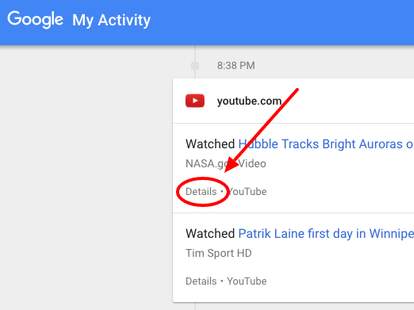The image showcases a "Google My Activity" screen with a white header against a blue background. Below this, there's a card for a YouTube video featuring an image of the Dalai Lama titled "Hubble Tracks Bright Auroras" in blue text, credited to NASA. 

A highlighted section with a red circle and an arrow pointing from the top emphasizes this card. Next to it, another card presents the video "Patrick Lane's First Day in Winnipeg" in blue, attributed to "Team Sport HD" in gray. The screen also includes additional smaller details like a bullet point followed by the word "YouTube" and an annotated box to the right of each video listing. 

The dialog box with a white background displays these activities, set against a gray backdrop on the left. Notably, above the detailed entries is the number "838." All text in the first line shares the same size but varies in color, while the fonts for NASA and Team Sport HD differ slightly. The "Details" text is slightly smaller than the other text elements.